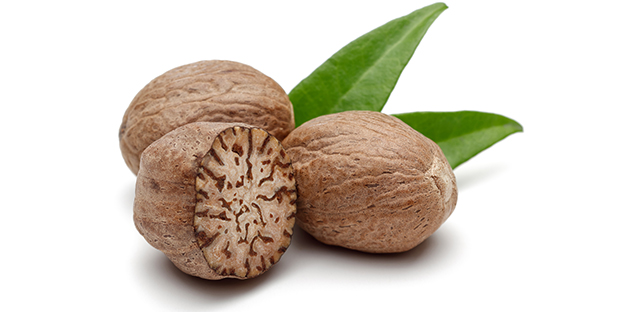The image is a highly detailed and bright color photograph of three nutmegs set against a stark white background. The foreground features two whole, elliptical-shaped nutmegs with brown, chestnut-colored shells. One is situated slightly higher on the left and the other lower on the right, both oriented horizontally. In front of these, a third nutmeg is cut in half, revealing its intricate inner structure composed of light brown and beige segments. The background hosts two green, triangle-shaped leaves, providing a striking contrast to the nutmegs. The overall clarity of the image is exceptional, with every detail of the nutmegs and leaves prominently visible.